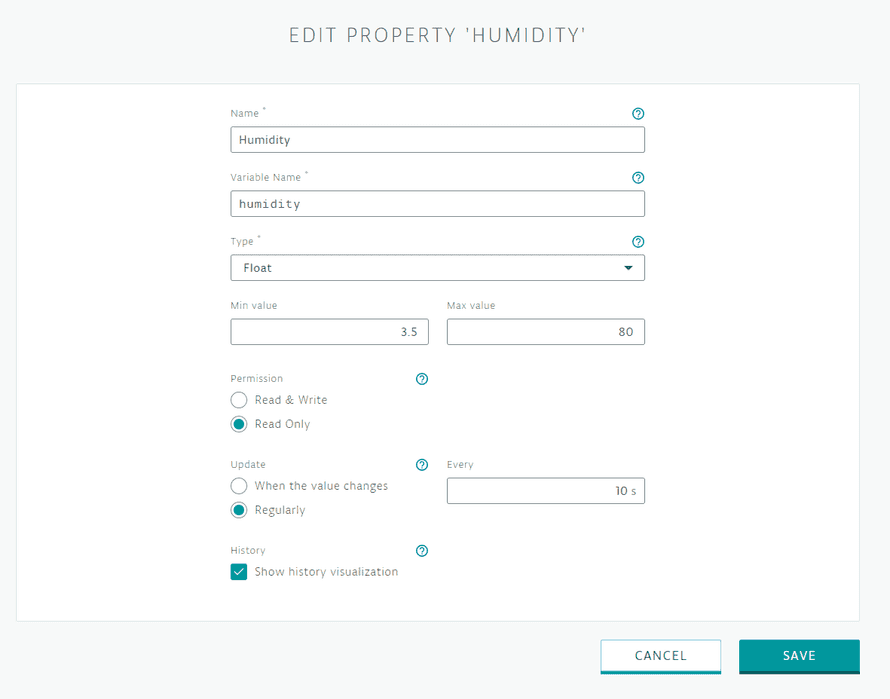The image depicts a section of a computer screen showing a detailed interface for editing properties related to humidity. At the top of the interface, a gray box contains the text "Edit Property," and a labeled section titled "Humidity." Below this header, there are multiple input fields and settings options.

1. **Name Field**: The top field is labeled "Name," currently filled with the text "Humidity." A teal-colored question mark icon at the end of this row offers additional help information.

2. **Variable Name Field**: Directly below, a field labeled "Variable Name" contains the text "humidity" in lowercase. Another teal-colored question mark icon is present at the end of this row for further assistance.

3. **Type Field**: This section is followed by the "Type" field, where the option "Float" has been selected.

4. **Value Constraints**: Next are the parameters for minimum and maximum values, specified as "Min Value 3.5" and "Max Value 80."

5. **Permission Settings**: Further down, there's a configuration for permissions, offering the choices "Read and Write" or "Read Only," with the latter currently selected.

6. **Updates Section**: This section discusses update settings, offering options for when to update values. The option "Regularly" is selected over "When the value changes."

7. **History Visualization**: At the bottom, there's an option to enable history visualization, marked with a checkbox labeled "Show History Visualization" that is currently checked. Adjacent to this setting, an input box labeled "Every" is filled with the value "10 S," indicating the interval for history updates in seconds.

Overall, the screen provides an extensive and customizable interface for managing humidity property settings, allowing the user to specify naming conventions, data types, value ranges, permissions, update frequencies, and visualization preferences.